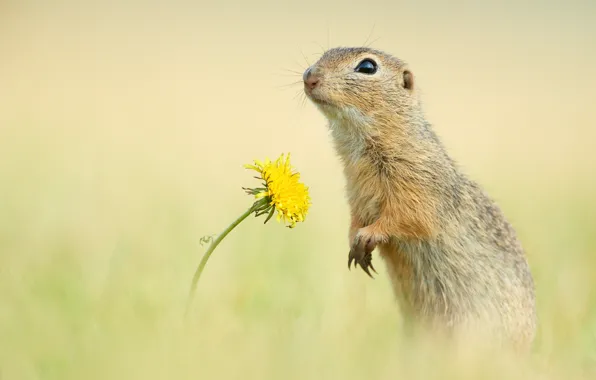In this captivating image, a sweet little groundhog is the main focus. He stands upright on his hind legs, with his front paws adorably folded across his chest, showing off his sharp claws. His glossy, teardrop-shaped eye gazes to the left at a bright yellow dandelion in full bloom, which stands almost as tall as he does. The groundhog’s fur is a pleasant mix of tan, brown, and gray with occasional dark spots, showcasing a natural gradient of colors. His small pink nose and fanned-out whiskers add to his charming appearance, while his tiny ears and glassy black eye lend him an inquisitive look. The background of the photo is beautifully blurred, consisting of light yellow and green hues that subtly frame the scene, creating a soft, dreamy atmosphere. The grass near the foreground is also blurred, bringing the sharply focused groundhog and the vibrant dandelion into even clearer relief.